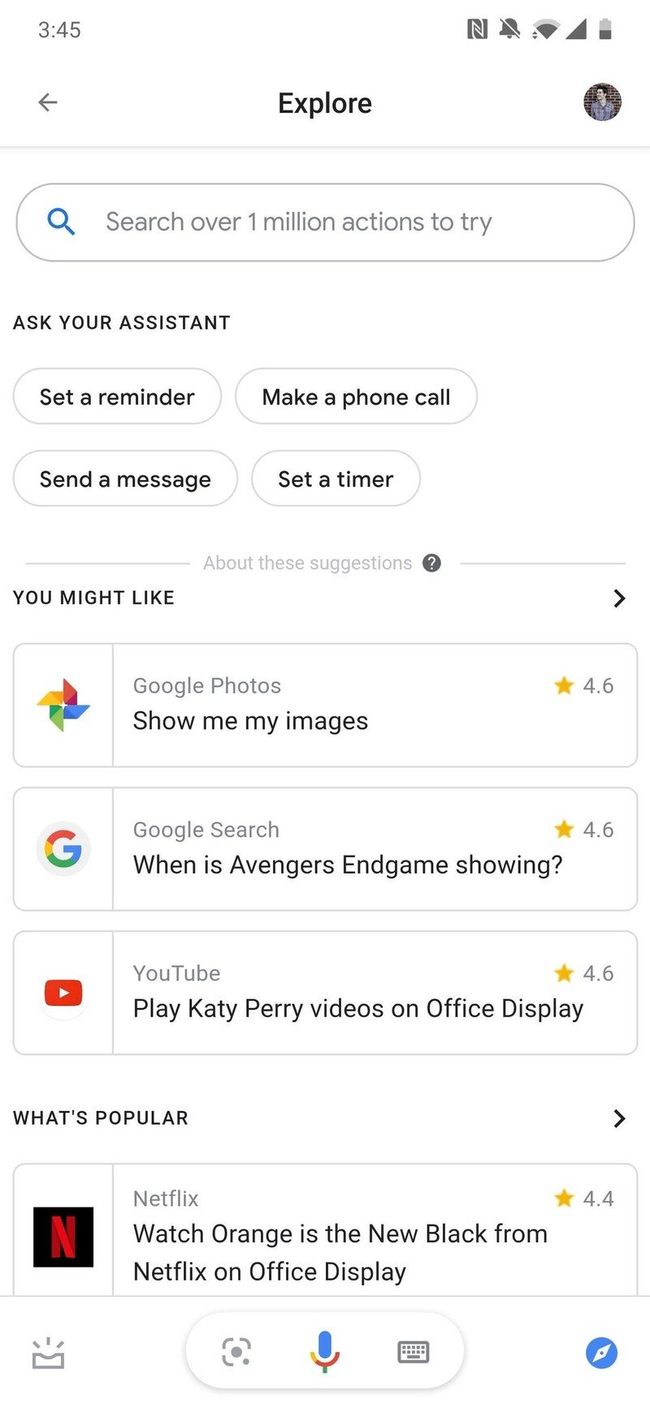The mobile screenshot in the image presents an interface rich with features and options for interaction. In the top left corner, there is a back arrow labeled "Explore" next to a small, unclear profile picture of a person. A search bar dominates the upper section, inviting the user to "Search for over 1 million actions to try" with a small blue magnifying glass icon to its left.

Following the search bar, there are several interaction options displayed as buttons: "Ask your assistant," "Set a reminder," "Make a phone call," "Send a message," and "Set a timer." Below these buttons, a gray line with the text "About these suggestions" is accompanied by a gray circle containing a white question mark.

Further down, under the section "Suggestions you might like," there are various action buttons: 
1. "Google Photos" with a 4.6-star rating and the prompt "Show me my images," featuring the Google Photos logo.
2. "Google Search" with a 4.6-star rating and the query "When is Avengers Endgame showing?" accompanied by the Google logo.
3. "YouTube" with a 4.6-star rating, offering to "Play Katy Perry on office display," showing the YouTube logo.

To the right of these buttons, an arrow suggests more options. Another section titled "What's popular" follows, showcasing:
1. "Netflix" with a 4.4-star rating, offering to "Watch Orange is the New Black on office display," highlighted by the Netflix logo.

At the bottom of the interface, there are four distinct icons:
1. A box with lines coming off it.
2. A circular icon within an incomplete box.
3. A multicolored microphone symbol, blending blue and red.
4. A blue compass.

The layout is thoughtfully organized to offer a wide range of actions and suggestions in a visually accessible manner.